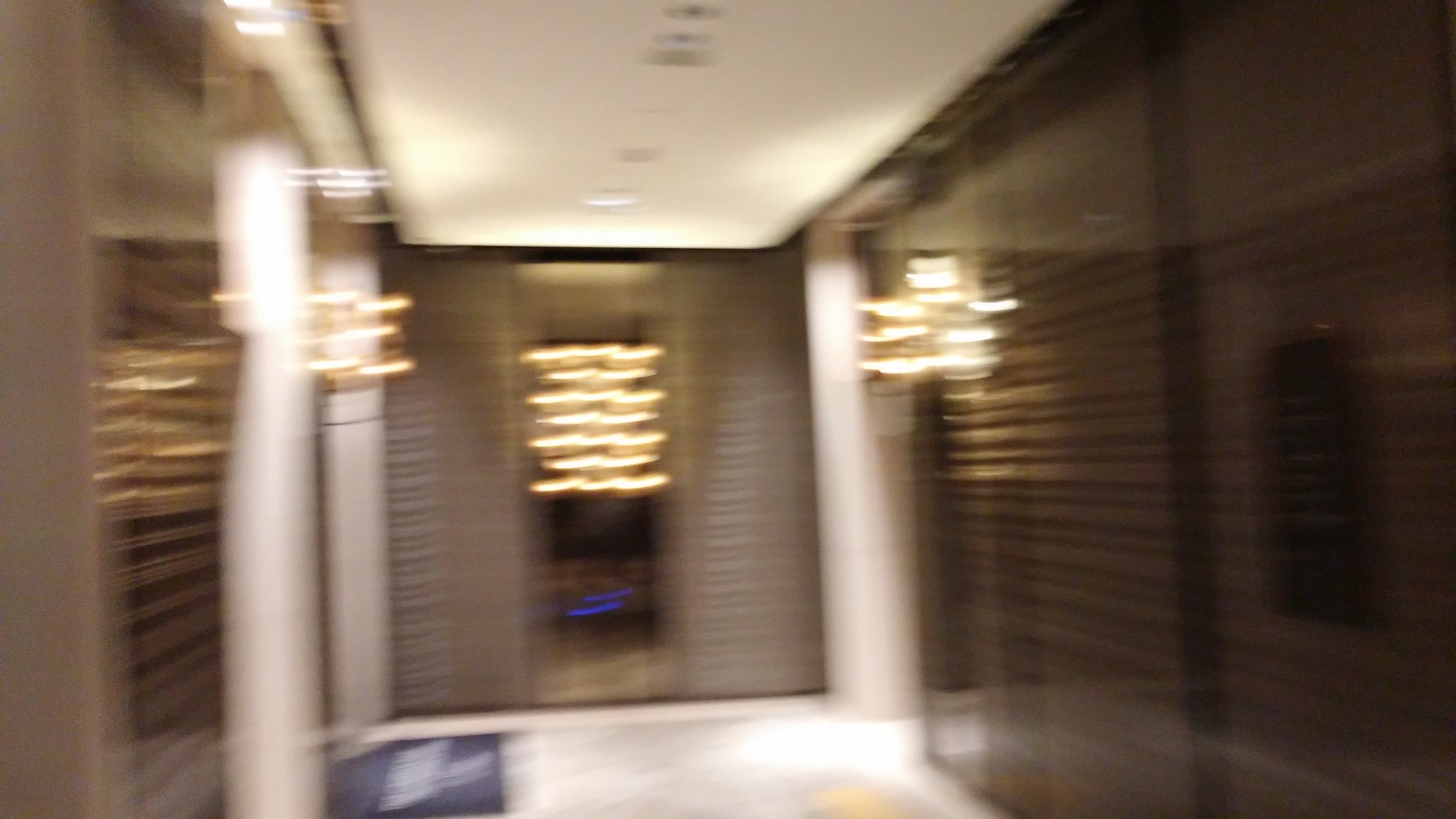This blurry photograph depicts the interior of a building, likely a lobby or an elevator area. The white ceiling features built-in, round downlights. Prominent in the image are reflective wall surfaces with a predominantly brown hue, and a mirror in the center of the back wall flanked by strands of white lights moving horizontally. Both sides of the image show large white pillars. On the left side, adjacent to a brown section of wall, there is a white wall and possibly a cluster of mailboxes. The middle right of the image showcases another white pillar leading into an opening. Beneath this pillar, you can spot a black structure, potentially an elevator control panel. The white floor contrasts sharply with a blue floor mat, also noticeable near the bottom left corner, bearing indistinct white text. The image is characterized by numerous lines of light, likely from long exposure, creating a squiggle effect across the scene.